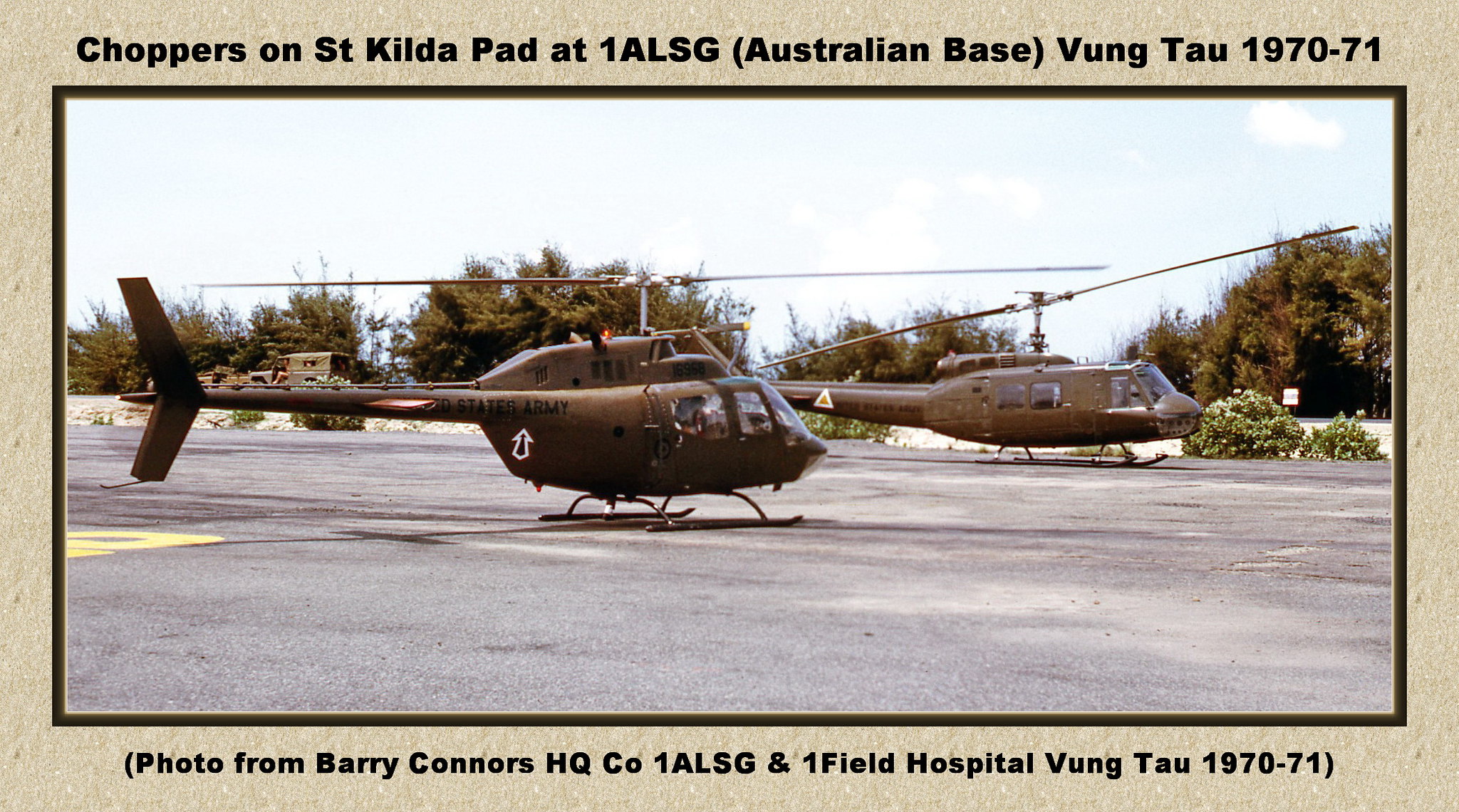This photograph, taken during the Vietnam War between 1970-1971, showcases two military helicopters stationed on St. Kilda's Path at the 1st Australian Logistic Support Group (1ALSG) base in Vung Tau, South Vietnam. The helicopters, painted in a brown olive green color, are parked on a wide concrete landing strip that features distinctive yellow lines. The scene is set against a backdrop of large trees and bushes, providing a sense of the base's surrounding environment. The photograph comes from Barry Connors, of the Headquarters Company, 1ALSG and 1 Field Hospital, and highlights the Australian military presence and operations during this period. A tan border frames the image, adding to its historical documentation.